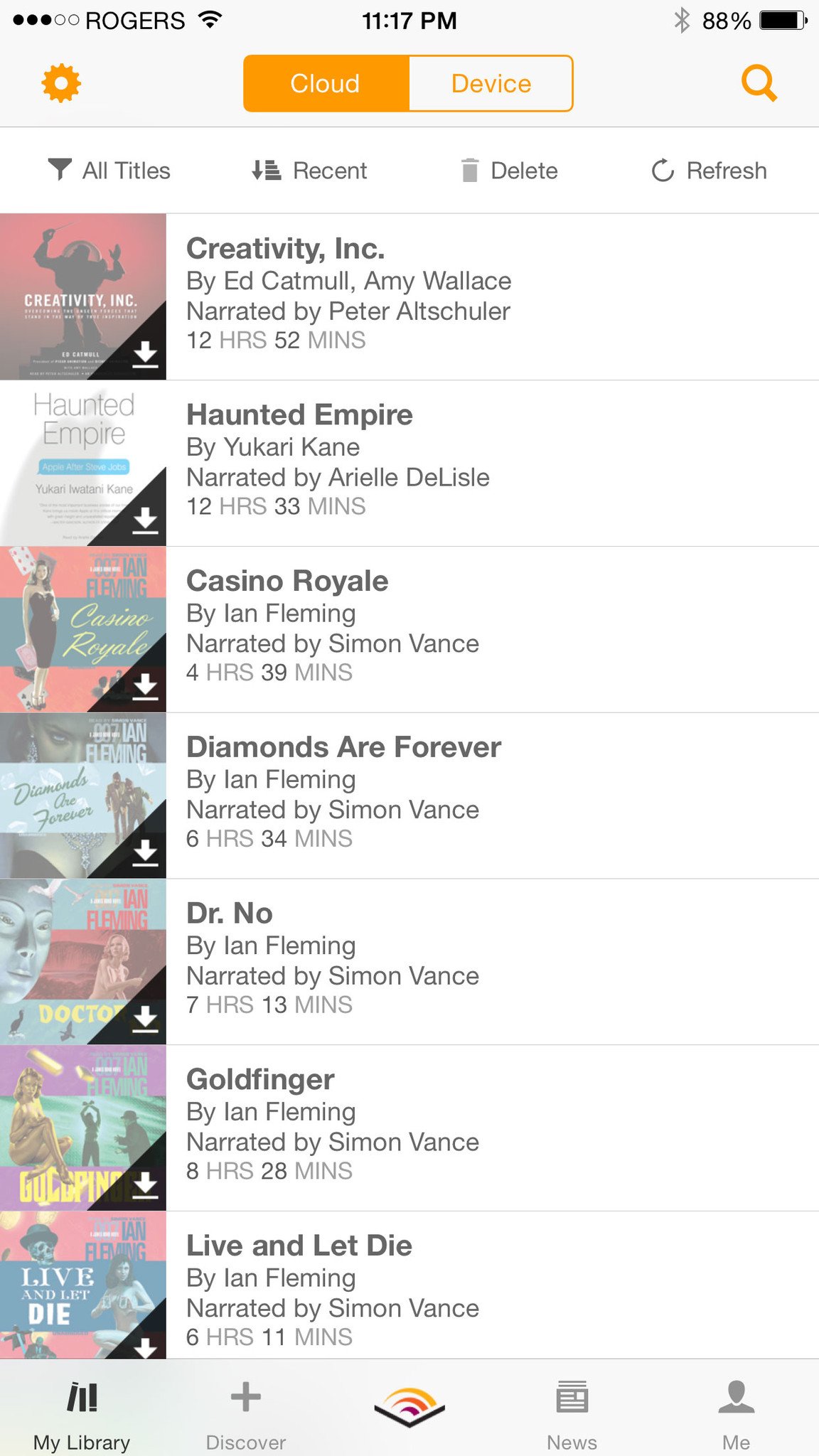**Descriptive Caption:**

The image is a screenshot from a tablet or smartphone displaying various interface elements. At the top left, the signal strength is represented by five circles, with three filled in and two empty, indicating a partial signal. Adjacent to this is the word "Rogers," identifying the Canadian cellular service provider. The top right corner features a fully filled wireless signal icon, signifying strong Wi-Fi connectivity. Centered at the top is the time, stated as 11:17 PM in black text. Nearby, a grey Bluetooth symbol and an 88% battery indicator are visible.

Below these indicators, there is an orange gear icon. Two rectangular tabs, labeled "Cloud" and "Device," are also present, with "Cloud" highlighted in solid orange, indicating it is selected. To the right of these tabs is an orange magnifying glass icon, implying a search function. This section is set against a cream-colored background.

Centered on the screen is a large white rectangle containing multiple tabs without separation lines. The tabs include:
- A chalice icon with the text "All Titles."
- A staircase icon with a down arrow and the text "Recent."
- A trash can icon labeled "Delete."
- An arrow forming a loop, labeled "Refresh."

On the left side within this rectangle, there is a list of different audiobooks, each accompanied by their respective details:
1. **"Creative Inc"** by Ed Catmull (C-A-T-M-U-L-L) and Amy Wallace (W-A-L-L-A-C-E), narrated by Peter Altschuler (A-L-T-S-C-H-U-L-E-R), with a duration of 12 hours and 52 minutes.
2. **"Haunted Empire"** by Yukari Kane (K-A-N-E), narrated by Arielle DeLisle (E-L-L-E-D-E-L-I-S-L-E), 12 hours and 33 minutes.
3. **"Casino Royale"** by Ian Fleming, narrated by Simon Vance (V-A-N-C-E).
4. **"Diamonds Are Forever"** by Ian Fleming, narrated by Simon Vance, 6 hours and 24 minutes.
5. **"Doctor No"** by Ian Fleming, narrated by Simon Vance, 7 hours and 13 minutes.
6. **"Goldfinger"** by Ian Fleming, narrated by Simon Vance, 8 hours and 28 minutes.
7. **"Live and Let Die"** by Ian Fleming, narrated by Simon Vance, 6 hours and 11 minutes.

All mentioned books are part of the James Bond series by Ian Fleming.

At the bottom of the screen, icons and their descriptions are shown:
- Books icon in black silhouette with the caption "My Library."
- Gray plus icon with the label "Discover."
- An open book icon with bands of orange, red, and purple, possibly representing Audible.
- Newspaper icon labeled "News."
- An icon combining a circle and crescent moon labeled "Me," indicating a user profile section.